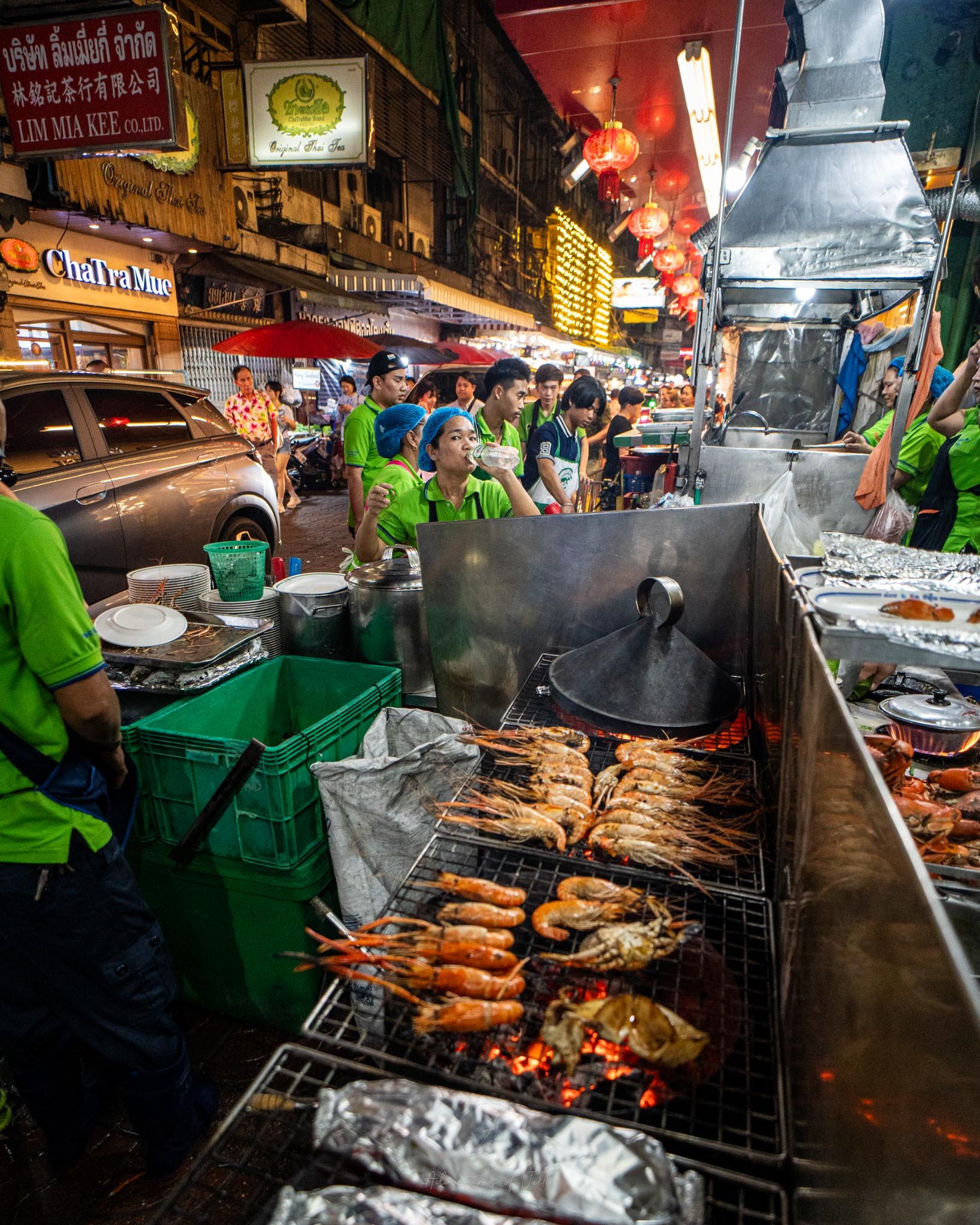In this bustling outdoor marketplace, presumably located in Thailand as indicated by the prominent Thai text on some signs, we see a vibrant and crowded street scene. The center of the image is marked by a silver panel surrounded by a distinctive black and silver grid, comprising four panels. Below this grid, a red glow emanates, adding a touch of vivid color to the scene. A row of six orange shapes can be observed on the center panel, with a shiny, silver foil-like object in the foreground. Beige and gray items are visible over the red glow, while a cream-colored long shape with hair protrudes from the adjacent panel.

On one side of the street, people clad in neon green shirts busily tend to a large grill, where jumbo shrimp and possibly crab are being freshly grilled. Nearby, a green bin can be seen along with a black triangular dome. The street itself is bustling with activity, featuring a mix of pedestrians, a car, and numerous storefronts. Some of these signs include names such as Chatramuc and Limmyakikol Limited amidst a flurry of other signage and a variety of storefronts with potentially apartments above.

Above this vibrant street, red lanterns dangle from a covered area, adding further to the atmosphere. The left side of the image shows a collection of busy, colorful elements in brown, red, and yellow hues, adding to the lively and chaotic feel of this quintessentially Thai marketplace.